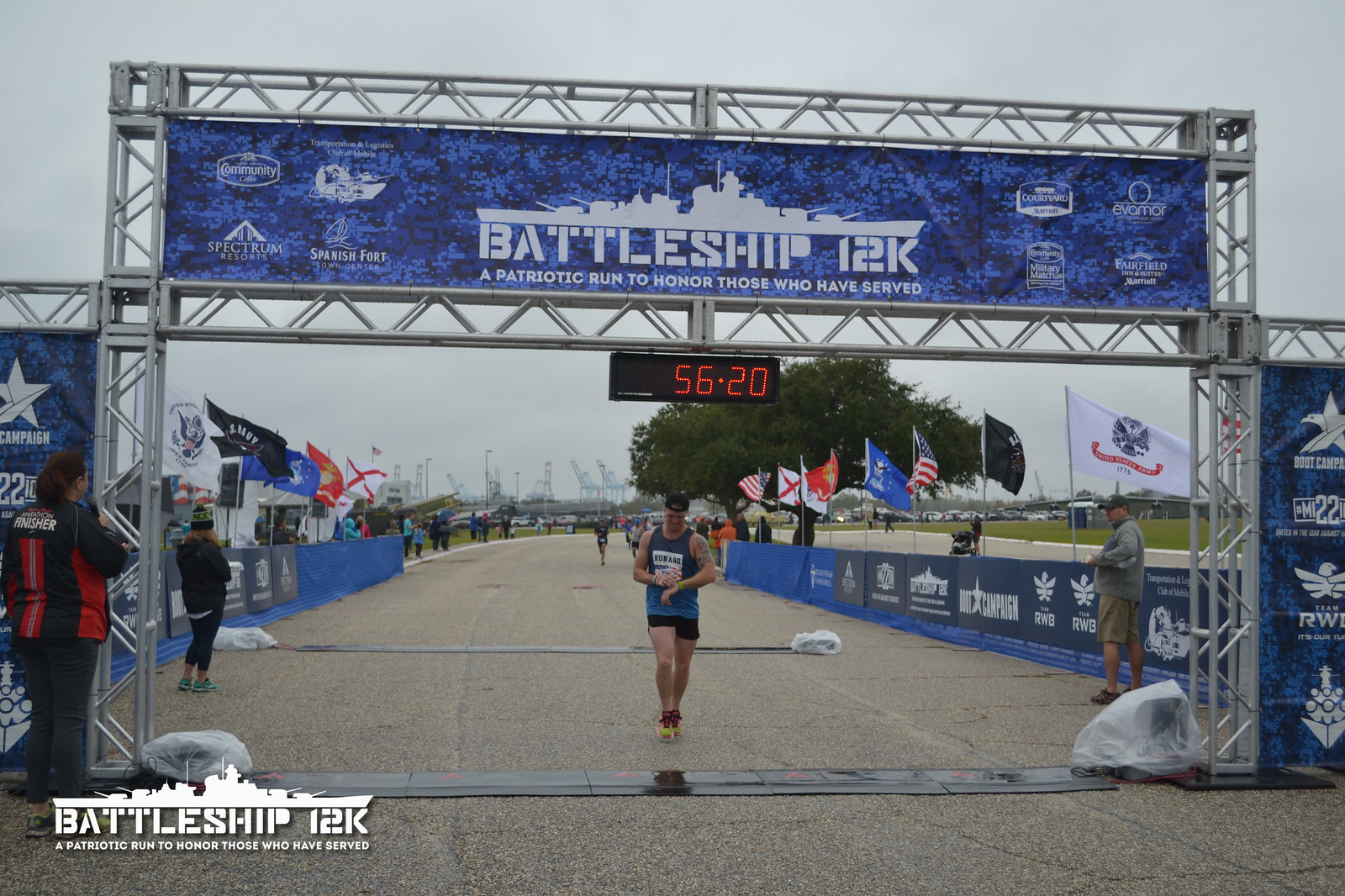In this image, a male runner is crossing the finish line of the Battleship 12K race, a patriotic event honoring veterans. The finish line features a blue banner overhead with "Battleship 12K" emblazoned on it, accompanied by a graphic of a fighter ship and various sponsor logos, including Community Coffee, Spectrum Resorts, Transportation and Logistics, Club of Mobile, Spanish Fort Town Center, Courtyard Marriott, and Fairfield Inn. The runner wears a blue tank top, black shorts, and a black baseball cap, and has visible tattoos. He is glancing at his watch as he completes the race in 56 minutes and 20 seconds, as displayed in red digits above him. The race course is a gravelly road lined with numerous flags from different countries, including the United States, U.S. Navy, U.S. Army, and U.S. Marine flags, creating a patriotic atmosphere. Spectators are positioned on both sides of the course, watching the runner's finish. The sky is overcast, adding a grey tone to the scene, and a sign at the bottom left corner reiterates the event name, "Battleship 12K," in white font.